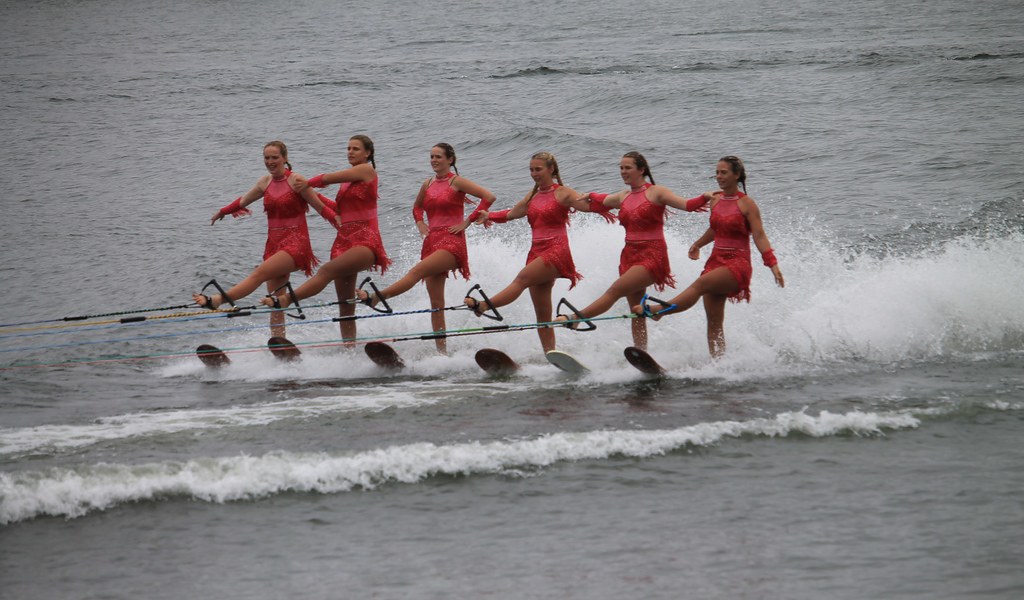In the photograph, six women are executing a synchronized water skiing performance. They glide in a straight line, each with their arms outstretched, hands resting on the shoulders of the skier next to them. Adorned in matching red, sleeveless dresses that resemble crop tops and skirts with fringes, they exude a sense of unity and grace. Each performer also wears red bracelets on their wrists, adding a touch of cohesion to their vibrant ensembles. Their left legs are extended ahead, with their feet gripping the handles of the jet ski ropes, while their right feet remain anchored on individual skis. Against the backdrop of a churning, white wake, the water beneath them appears as a grayish-green expanse, indicating a lake or ocean setting. The women's hair is uniformly tied back, and they look to be anywhere from 18 to 30 years old, though their exact ages are obscured due to the distance of the shot. The overall scene captures the thrill and precision of the sporting event, highlighting the impressive skill involved in their synchronized routine.